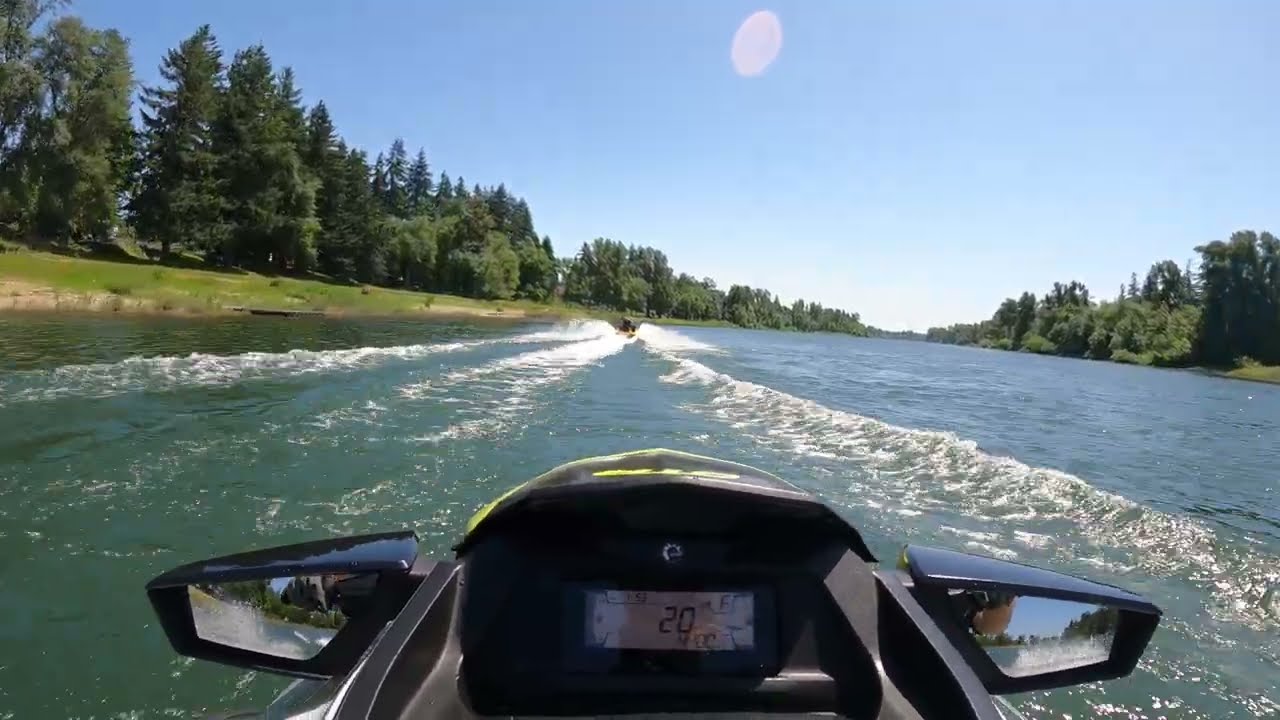The photograph captures a vibrant scene set on a serene body of water, possibly a lake or a slow-moving river, framed by grassy banks and abundant evergreen trees on both sides. The sky above is a clear blue, with a few clouds near the horizon. At the forefront, the image partially shows a black and yellow jet ski, specifically its front panel featuring an LCD display indicating a speed of 20 miles per hour. Side mirrors attached to the jet ski reflect the rider's arms and hands gripping the throttle. The water, colored a seafoam green, showcases waves created by another jet ski ahead of the primary one, cutting through the water and leaving a distinct wake that almost forms a watery pathway. This preceding jet ski is also present in the distance, reinforcing the sense of motion and high-speed activity amidst the clear and bright daytime setting.